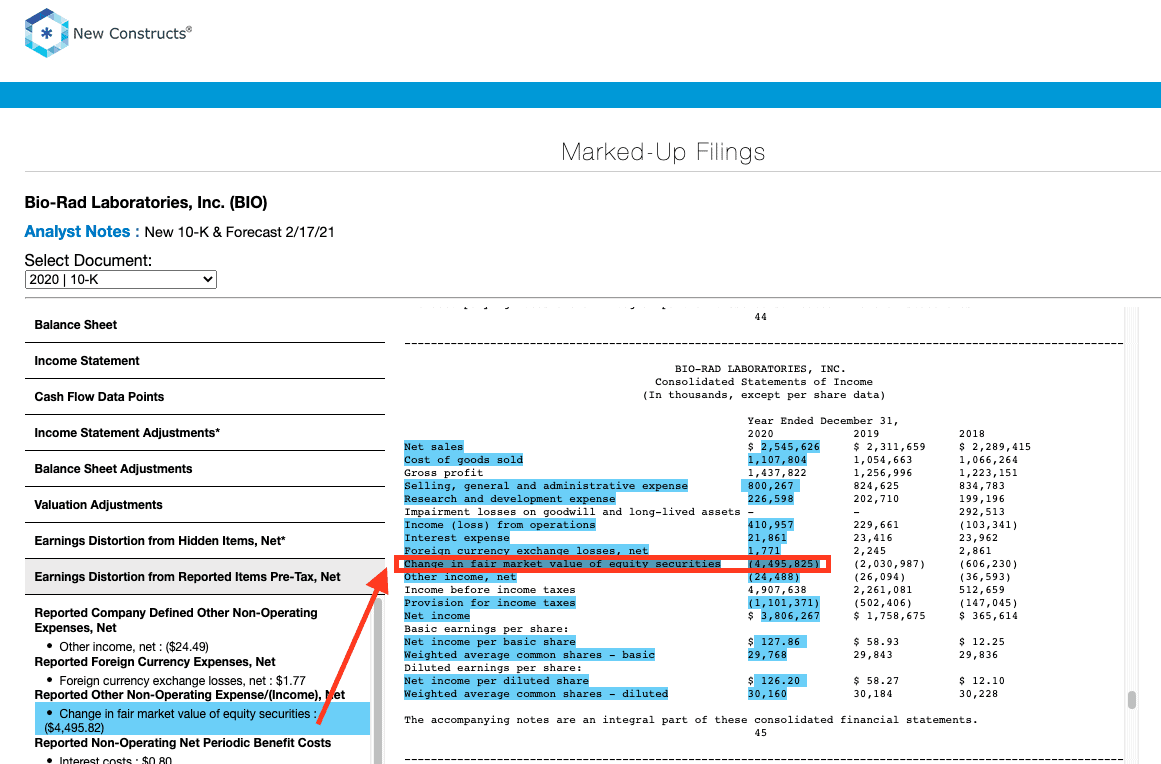The image depicts a detailed financial analysis for Bio-Rad Laboratories Inc. on February 17, 2021. Key elements include new constructs registered and marked-up filings, encompassing the latest 10-K report and forecast. The select document outlines crucial financial statements — the balance sheet, income statement, and cash flow. Data points are meticulously highlighted, detailing income statement adjustments, balance sheet adjustments, and valuation adjustments. It further breaks down earnings distortions from both hidden and reported items, pre-tax net income, and various other financial metrics. Specific figures include $24.49 listed under other non-operating expenses net, and $1.77 corresponding to reported foreign currency exchange losses net. This comprehensive analysis captures other non-operating expenses and income, encapsulating the company's financial health and projections.